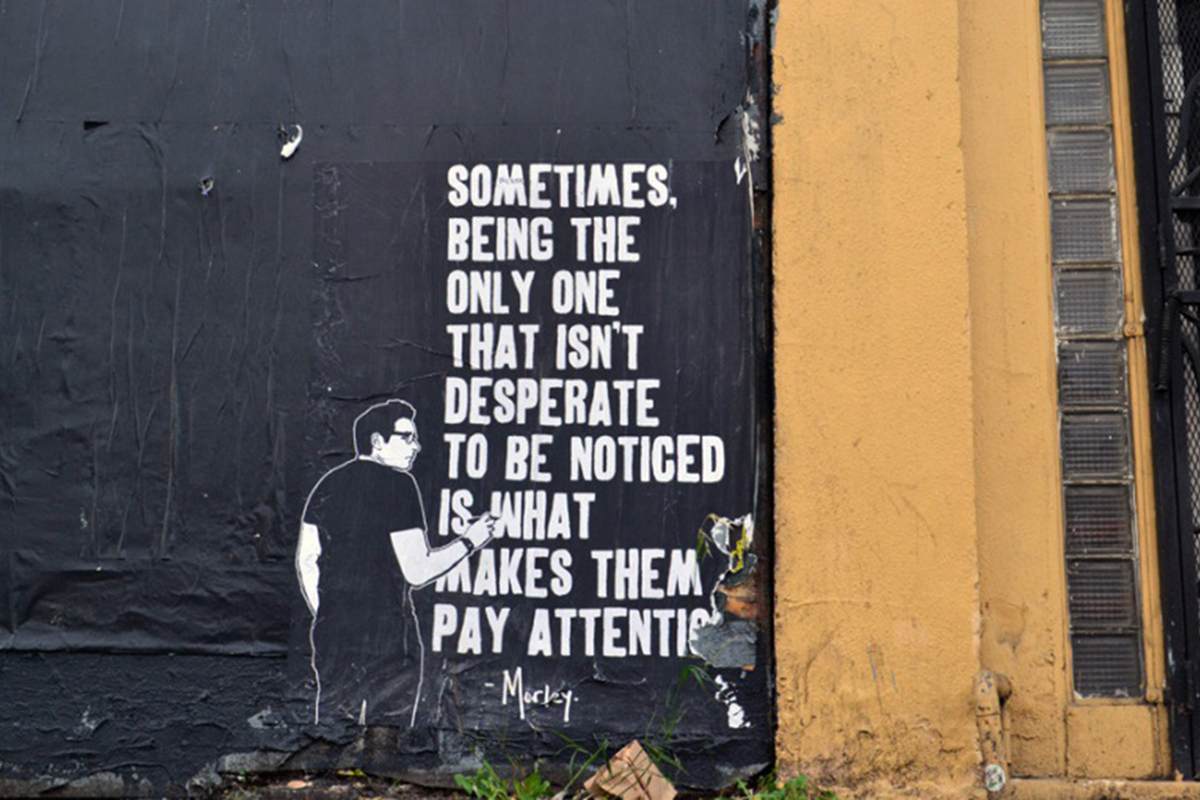This photograph captures a piece of street art painted on an outdoor wall, presumably in Europe. The mural features a profound message in bold white letters against a black background, reading: "Sometimes being the only one that isn't desperate to be noticed is what makes them pay attention." To the right, the scene is anchored by an industrial-looking tall orange column and large glass block windows with black mesh fencing. The artwork includes a detailed depiction of a man seen in profile, dressed in all black with white accents outlining his figure. He wears glasses and a watch, and his dark hair contrasts with his white face and arms. The man appears to be in the act of writing or drawing the quoted message on the wall, holding a paintbrush in his right hand. The bottom of the photograph shows a strip of grass and some scattered trash, adding to the gritty urban atmosphere. The artwork is signed with the name "Maki" or "Marley," suggesting the identity of the artist.